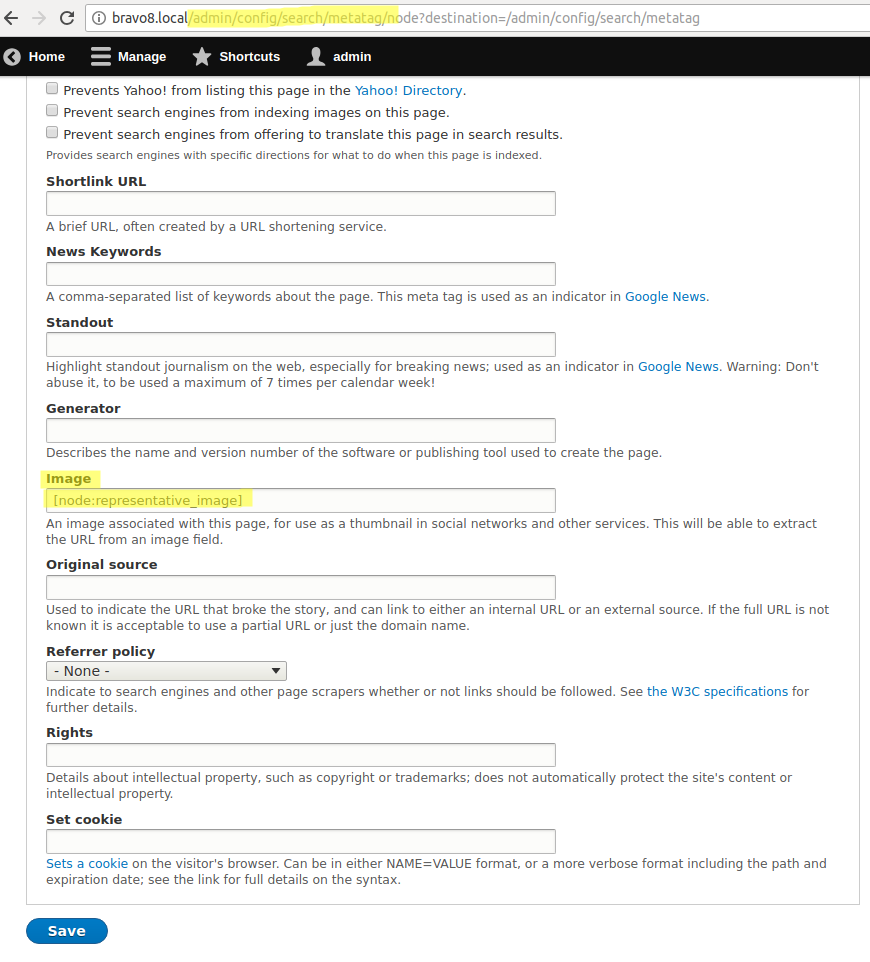The image depicts a registration form with several interactive elements and instructions for setting up webpage visibility and metadata. At the top, a left-facing arrowhead with a gray circular background and white text labeled "Home" appears. Adjacent to it are three horizontal lines representing a dropdown menu, followed by "Manage" in white text. 

Next, a gray star icon labeled "Shortcuts" in white text is visible. This is followed by the silhouette of a person in gray, and next to it, "Admin" in white text.

Below this header, there are three unticked checkboxes with the following options:
1. Prevents Yahoo from listing this page in the Yahoo directory (with "Yahoo directory" in blue, indicating a clickable link).
2. Prevent search engines from indexing images on this page.
3. Prevent search engines from offering to translate this page in search results.

Further down, a bold label reads "Short Link URL" with an empty field underneath. Below the field, in light gray text, a description reads, "A brief URL, often created by a URL shortening service."

Next, a section titled "News and Keywords" in bold black text appears, followed by an empty space for input. Below this, in a smaller gray font, the instruction reads, "A comma-separated list of keywords about the page. This meta tag is used as an indicator in Google News," with "Google News" in blue, indicating a clickable link.

Another section labeled "Standout" in bold text follows, featuring an empty input field. Beneath it, smaller, gray text advises, "Highlight standout journalism on the web, especially for breaking news used as an indicator in Google News. Warning: don't abuse it. To be used a maximum of seven times per calendar week!"